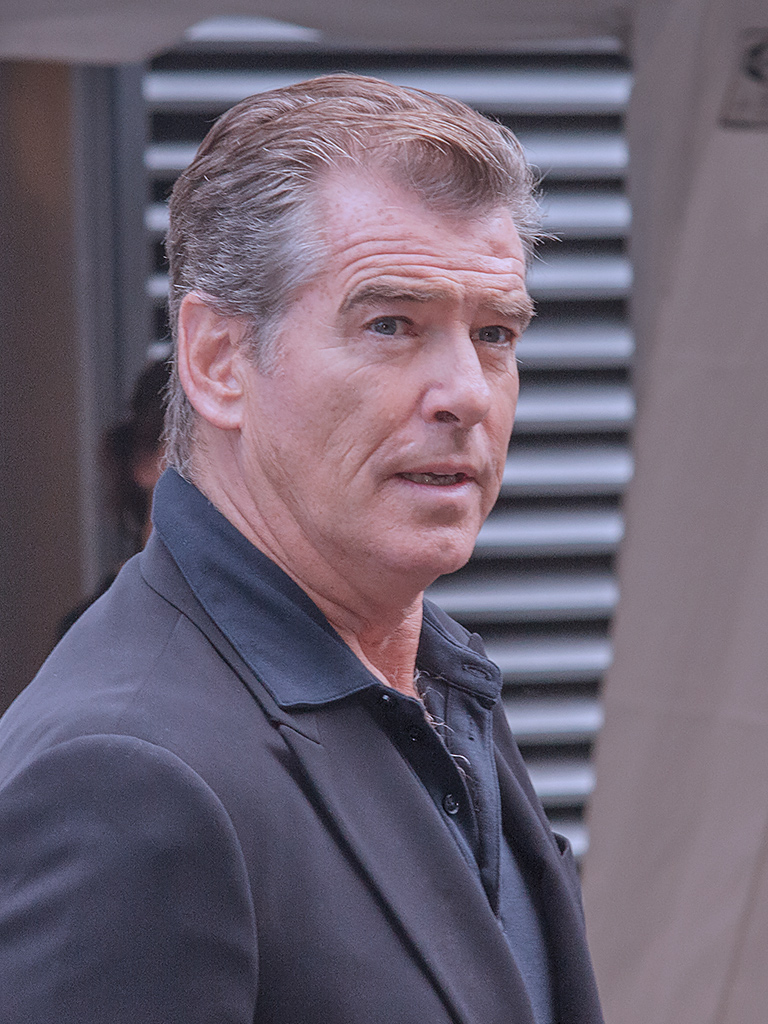This detailed photograph captures a middle-aged man, presumably a movie or television star, standing outside against a backdrop of metal shutters and a wall. His attire includes a sleek black jacket over a partially unbuttoned black button-up shirt, revealing a glimpse of chest hair. The man, with his face lined with noticeable wrinkles, features slicked-back gray hair and a receding hairline. His eyebrows are bushy, blue eyes look slightly off to the side, and his mouth is ajar without any distinct facial expression. Adding to his polished yet rugged appearance are sideburns running halfway down his ears. Positioned to the right with his body, he turns his head towards the camera. In the background, there's a faint outline of a woman with dark hair, adding another layer of context to the scene.